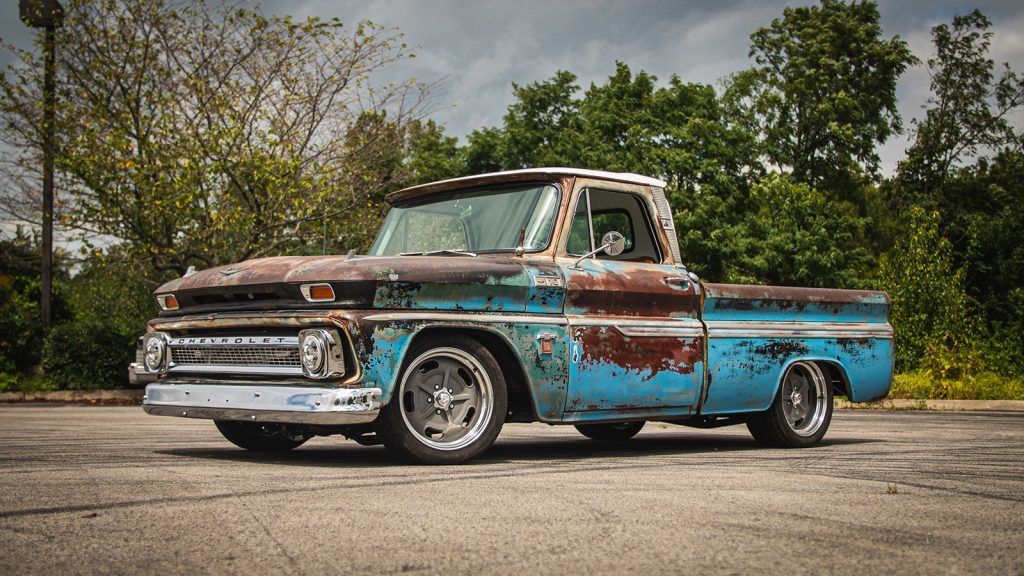In this photograph, we see an old, rusty Chevrolet pickup truck, possibly from the 1950s or 1960s, parked on a concrete asphalt area with a gray curb. The vehicle, which once boasted a light blue paint job, is now predominantly covered in rust and patina, presenting a nostalgic charm despite its weathered condition. The hood is almost entirely rusted, while the sides still hint at its original blue color amidst the extensive rust on the door and bed. 

The truck features a long, rectangular chrome grille with two round headlights and "Chevrolet" emblazoned on the chrome. The bumper is also chrome, adding to its classic appearance. The truck has four visible tires with silver rims and modest, possibly thicker tires than it originally came with, suggesting it might have been modified or well-maintained despite its aged exterior. 

The windows are down on the left-hand side, and a light pole is visible in the top left corner of the image. The background consists of dense green trees and bushes, contributing to a sense of abandonment. The sky above is gloomy and overcast, indicating an impending storm. The scene exudes a sense of nostalgia and resilience, capturing the enduring essence of a bygone era.